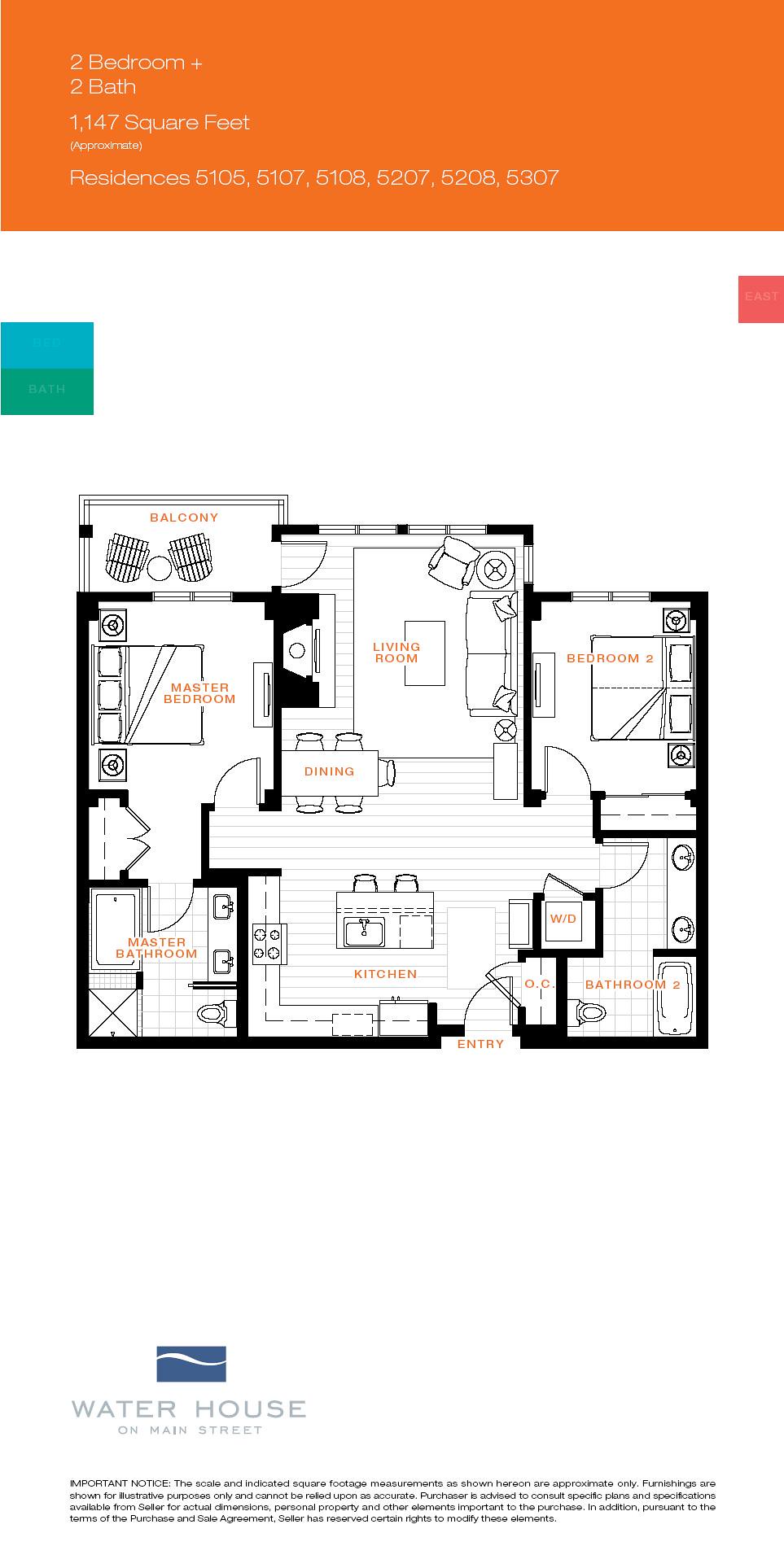This detailed floor plan depicts a 1,147 square foot, two-bedroom, two-bathroom apartment. At the top of the image, an orange band prominently displays the label "Two Bedroom Plus Two Bath | 1,147 Square Feet Approximate," alongside the residences numbered 5105, 5107, 5108, 5207, 5208, and 5307. Adjacent to this, on the right side, there's a small pink square subtly marked with the word "East" in light pink text.

Opposite this pink marker, there is a larger square featuring a blue band and a green band. The text on the blue band is illegible, but the green band clearly reads "Bath." The central floor plan reveals a nearly square layout with two bedrooms, two bathrooms, a living room, a dining area, and a kitchen, suggesting an apartment structure. The master bedroom includes a spacious ensuite bathroom, accessible through the closet area, while the second bedroom has convenient access to a bathroom located just outside its door. 

The apartment's entryway opens directly into the kitchen area. At the bottom of the floor plan, a blue rectangle with a white wave showcases the branding "Waterhouse on Main Street." Below this, a cautionary note in black text emphasizes that the scale and square footage are approximate and that furnishings are illustrative, thus advising purchasers to consult specific plans and seller specifications for precise details. The note further clarifies that the seller retains certain rights to modify these elements under the terms of the purchase and sale agreement.